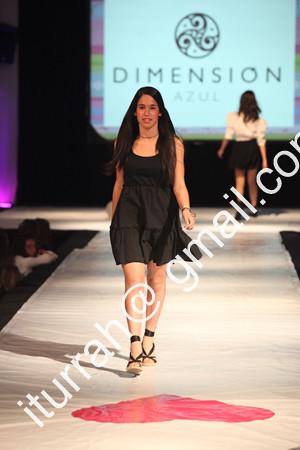In the image, a young woman with long dark hair is confidently walking down a white runway adorned with a large red heart near the end. She is dressed in a sleek, sleeveless black dress paired with black strappy sandals. Her outfit is complemented by a necklace, and her dark eyes gaze ahead. She is of Caucasian descent. Behind her, another woman with long black hair, wearing a white top and a black skirt, is seen walking in the opposite direction.

The background features a blue projection that reads "Dimension Azul," accompanied by a distinctive black logo, which appears to take an abstract form. To the left side of the catwalk, a seated child or small younger girl is intently watching the woman in the foreground. The scene is part of a modeling show, and diagonally across the image in white text is an email address, "iturah@gmail.com," although the ".com" is partly obscured.